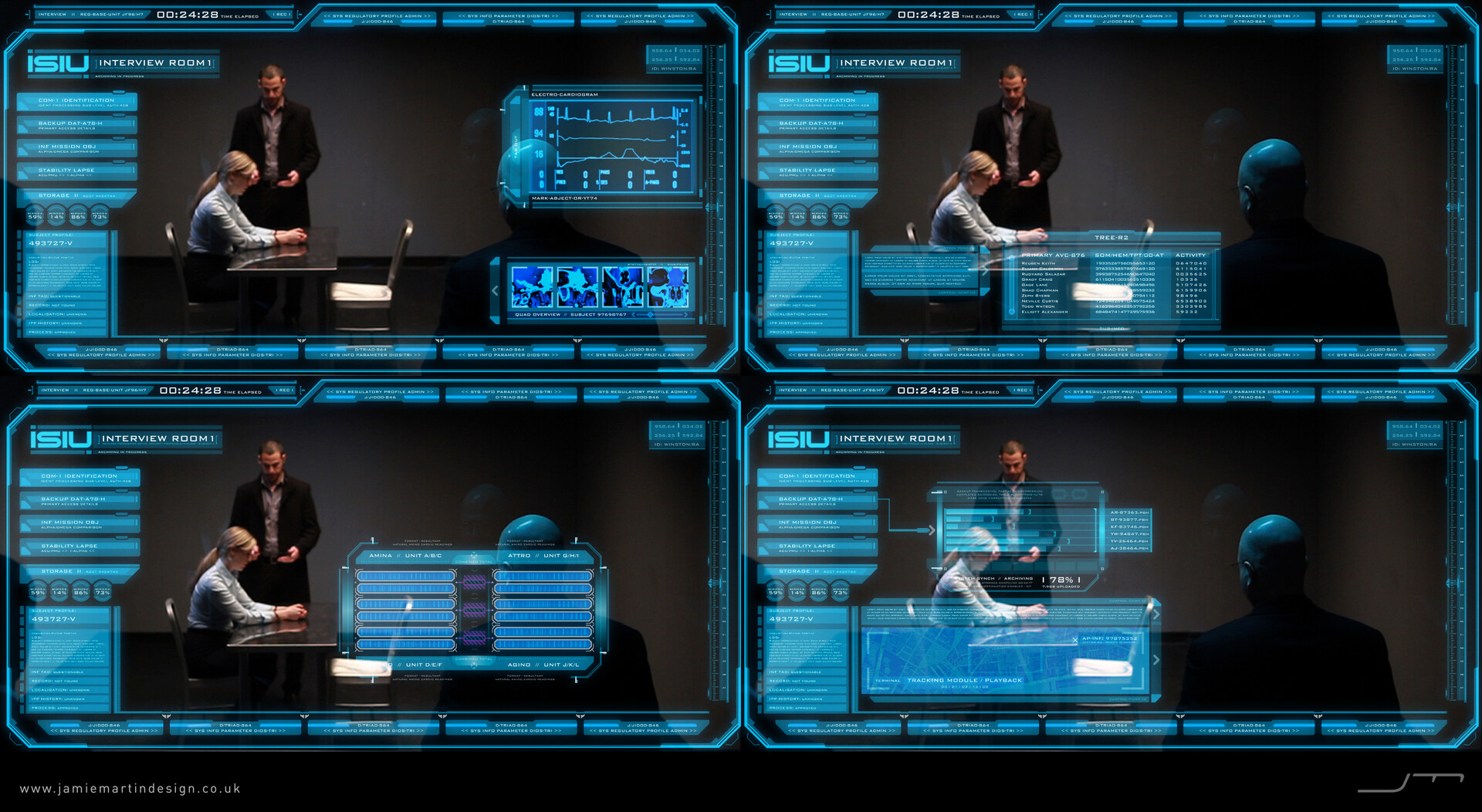This image is a composite of four horizontally aligned rectangular panels, resembling screenshots from a video game. Each panel is outlined with a thin blue border and displays a consistent scene with minor variations in graphical overlays. The scene features a woman with blonde hair tied in a ponytail, dressed in a white shirt and black pants or skirt, sitting at a gray table in an interview room. Standing over her is a man in a black suit, making gestures with his hands, seemingly in an interrogative stance. To the right, in the foreground of each panel, there's a bald man in a black suit viewed from behind. He appears to be observing the interaction through a glass. Each frame has "ISIU Interview Room 1" marked in the top left corner. The charts, graphs, and pop-up boxes in each panel differ slightly in position and content, with some containing lines and arrows pointing to various sections. There is also fine, unreadable print at the bottom of the panels and a website link reading "www.jamiesomething.gn.co.uk" on a solid black background. All four panels display a timestamp of "24:20" in the bottom corner.